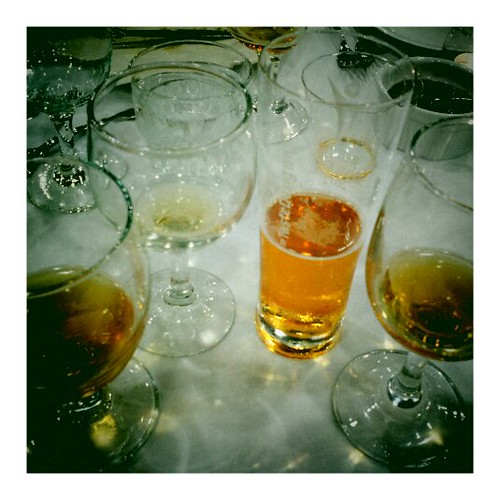This square-shaped color photograph captures an overhead view of a table set for a celebration, adorned with an assortment of barware. At the forefront, a brandy snifter and a goblet sit partially filled with dark amber liquor. Nearby, a tall, narrow tumbler—embellished with white, frosted Japanese writing—appears to hold beer, filled about three-eighths of the way. A wine glass and a margarita glass sit almost empty, catching the ambient light from above, which creates a striking interplay of reflections and shadows on the pristine white tablecloth. In the background, additional glassware, including chalices and goblets, along with place settings of white plates, forks, and spoons, lend a festive and elegant atmosphere to the scene. A metal pot or round bowl is also faintly visible, further suggesting a celebratory gathering.